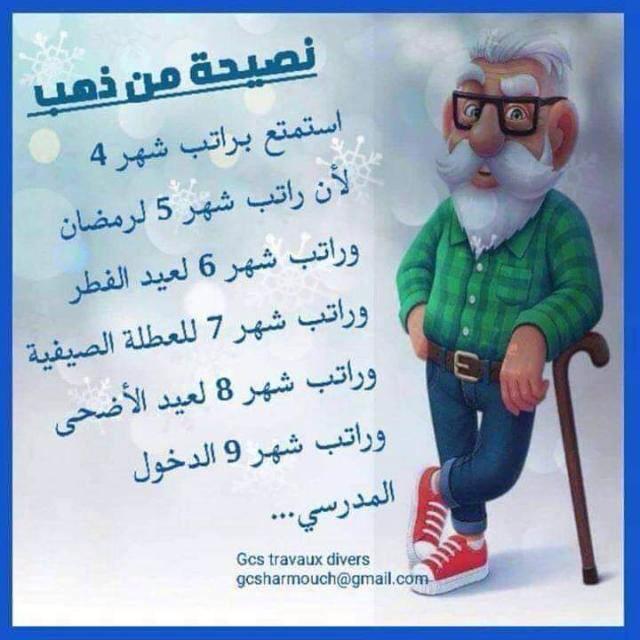This image showcases a card featuring a cartoon character of an elderly man with exaggerated features. The elderly man is characterized by his white undercut hair, thick white eyebrows, large ears, black-framed glasses, a prominent white handlebar mustache, and beard. He is dressed in a green plaid long-sleeve shirt, a belt, blue jeans with folded cuffs, and red sneakers. He is depicted leaning on a brown cane, with his legs crossed in an L shape. The background has a light gray snowy and spotlight pattern. On the left side of the card, there are six rows of Arabic text. Along the bottom center of the card, the text reads "GCSTRAVAUX DIVERS" followed by an email address: "gcsharmouche@gmail.com." The card has a blue outer border, contributing to its advertisement-like appearance.